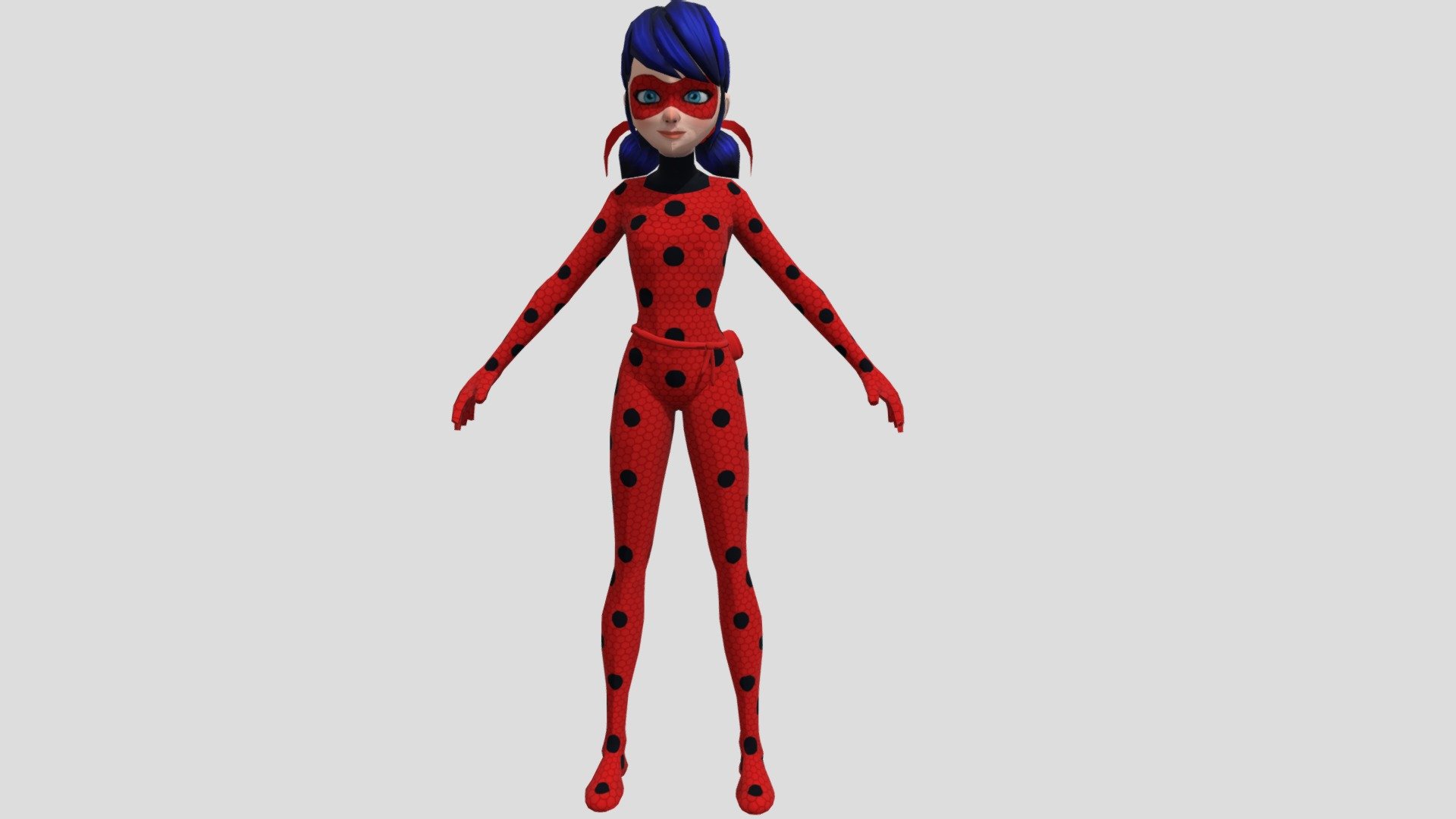The image is a rectangular screenshot, wider than it is tall, featuring a cartoon character named Ladybug prominently in the center. The backdrop of the picture is a solid gray or off-white. Ladybug is dressed in a striking red bodysuit adorned with black polka dots, covering her from neck to toes, including her feet. The suit has a honeycomb texture and resembles a matching set with a fitted long-sleeve top and pants.

She has navy blue hair styled in two low pigtails that rest on her shoulders, with subtle black stripes interspersed. Ladybug wears a distinctive red mask over her face, which features a figure-eight pattern around her bright blue eyes, and the mask ties into red ribbons above her hair, one ribbon on each side. Accentuating her appearance, she sports bright red lipstick.

Her black neck area seems to give the impression of a turtleneck, and she is captured facing directly towards the viewer with her arms slightly angled outwards, as if in a relaxed or neutral pose. A red tie or small bag is also noted around her waist, complementing her superhero attire.